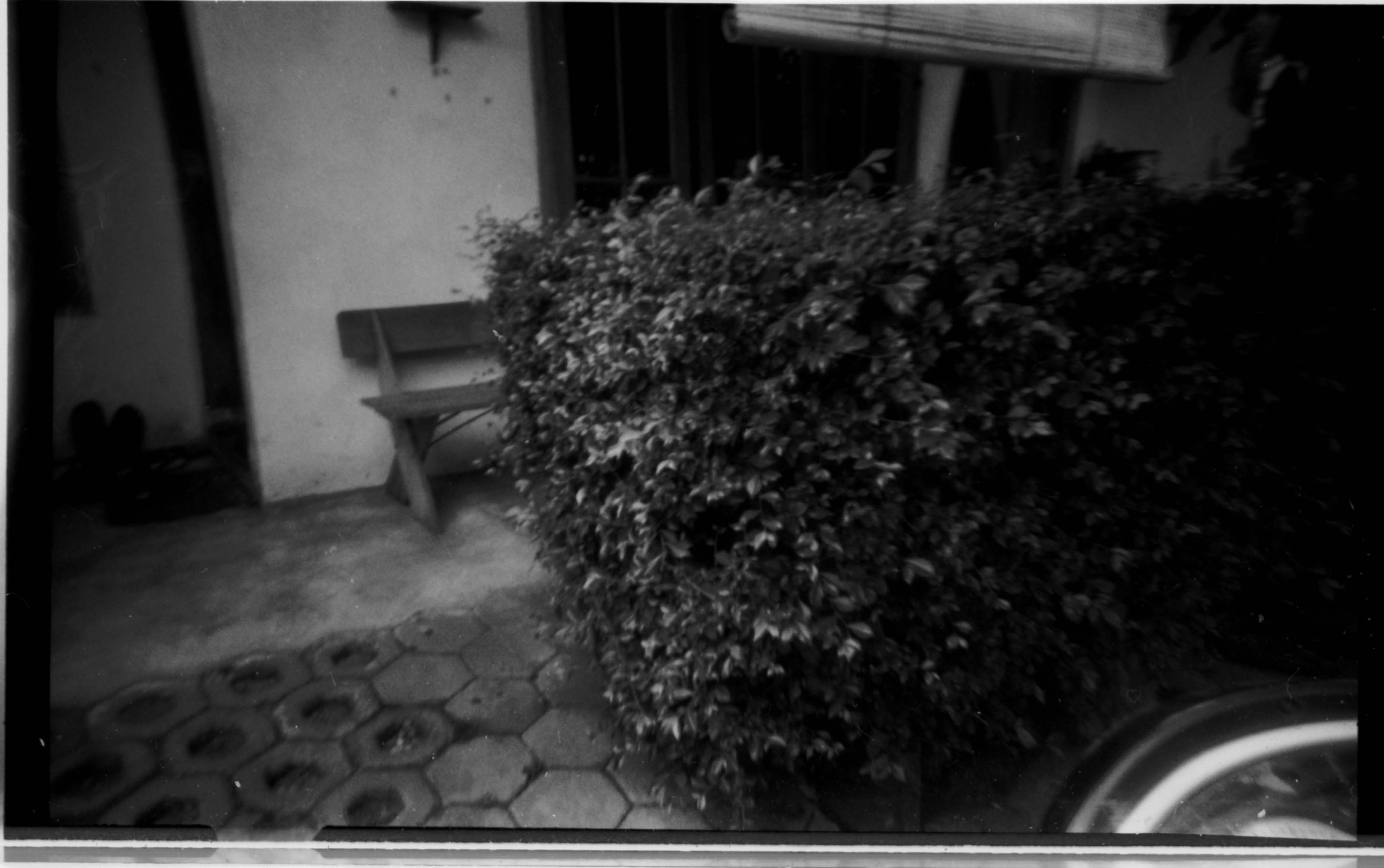This black and white nighttime photo depicts a detailed scene featuring various elements. Central to the image is a building with a distinctive white wall, possibly a house or store, framed by large shrubs that dominate the space. A wooden picnic bench rests against the building, partially obscured by the thick foliage. Above the bench, a light fixture is attached to the wall, illuminating part of the scene. To the right of the white wall is a section of glass, while to the left, an open doorway is visible. 

Foreground detail includes a walkway paved with numerous honeycomb-shaped bricks, some of which appear damaged with noticeable holes. The lower right corner of the image reveals what looks like a tire, possibly from a bicycle or car, lying next to the hedge. Additionally, the image features a sign emerging from the bush, though its text is unreadable due to the image's cropping. The contrast of textures, from the rough bricks to the smooth wall and the intricate details of the bush and bench, add depth to the nocturnal scene.